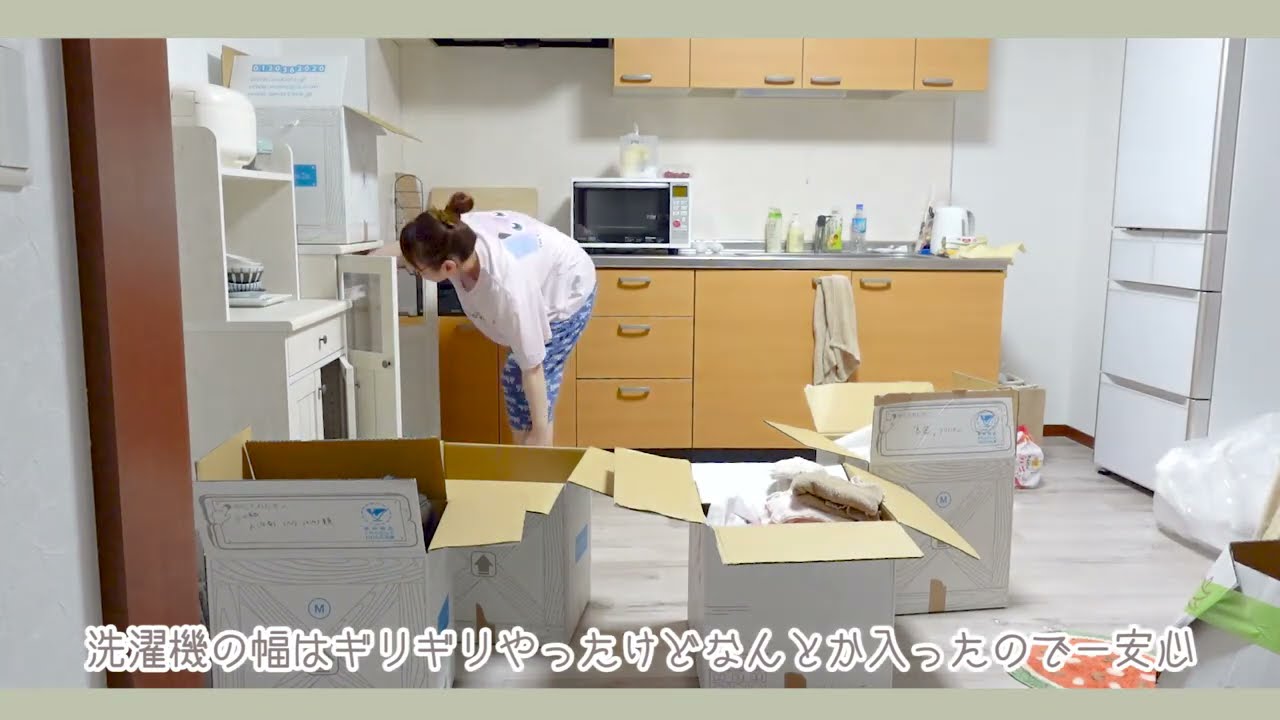A woman with brown hair tied in a bun is standing in a brightly lit kitchen area, wearing blue pants with white designs and a white shirt. Positioned on the left side of the image, she is hunched over, looking into an open white cabinet. The room is filled with various cabinets, some made of light wood with metallic handles, and others that are white, including a large white refrigerator with several drawers and compartments on the right. The countertop features a microwave or toaster oven beside a sink with beige cabinetry below, which includes three drawers on the left and two larger cabinets. Scattered across the vinyl-tiled floor are several open cardboard boxes, indicating a moving process. The kitchen exhibits a mix of utility and clutter, with cleaning accessories and a bottle of water visible. There is also some Asian script in white and gray at the bottom of the image, adding an international element to the scene.